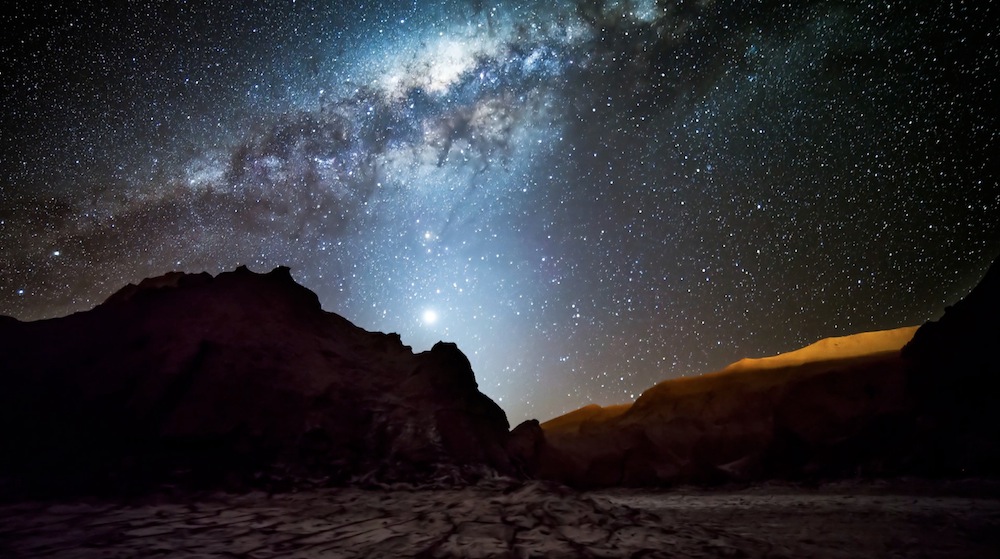This photograph captures a breathtaking nighttime desert landscape, featuring a dramatically craggy and jagged horizon occupying the bottom third of the frame. The arid, patchy ground leads up to rocky cliff-like hills and mountain peaks, which have an intense, blackened appearance in the night, except for a hint of golden illumination along the right side. Rising above this rugged foreground is an immense, extremely starry sky, brilliantly clear and unmarred by light pollution. Dominating the upper left corner is a mesmerizing band of the Milky Way, appearing as a glowing, nebulous streak with a distinctive white, cloud-like haze accented by dark, smoky lines. Millions of stars of varying brightness densely sprinkle the rest of the night sky, enhancing the majestic and serene atmosphere.